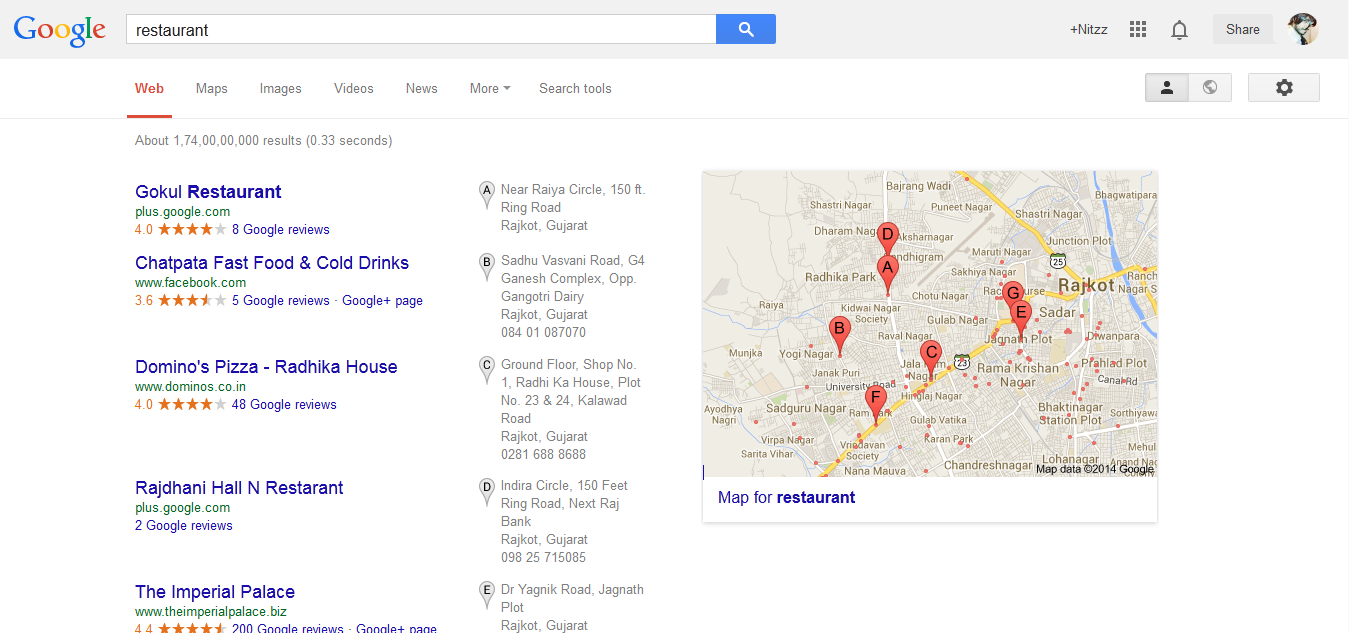The image appears to be a screen capture from a Google search for nearby restaurants, displayed either on a website or a tablet interface. At the very top is the Google header, featuring a search bar where the user has typed "restaurant," a search icon, and additional elements like the user's personal account, an option to share, and a button related to other Google services.

Below this gray header bar, there are navigation options labeled "Web," "Maps," "Images," "Videos," "News," and "More." The "Web" option is currently selected, displaying a list of restaurant search results near the user's location.

The search results include various restaurant names such as Gokul Restaurant, Chatpata Fast Food and Cold Drinks, Domino's Pizza, The Imperial Palace, and Rajan Hall Restaurant. Each restaurant entry provides detailed information such as the establishment's address, phone number, and links to reviews.

To the right of the search results, there is an interactive map displaying the locations of these restaurants. The map uses different alphabetical icons to mark each restaurant correspondingly.

The overall background is white, with no additional stylistic features or notable characteristics.